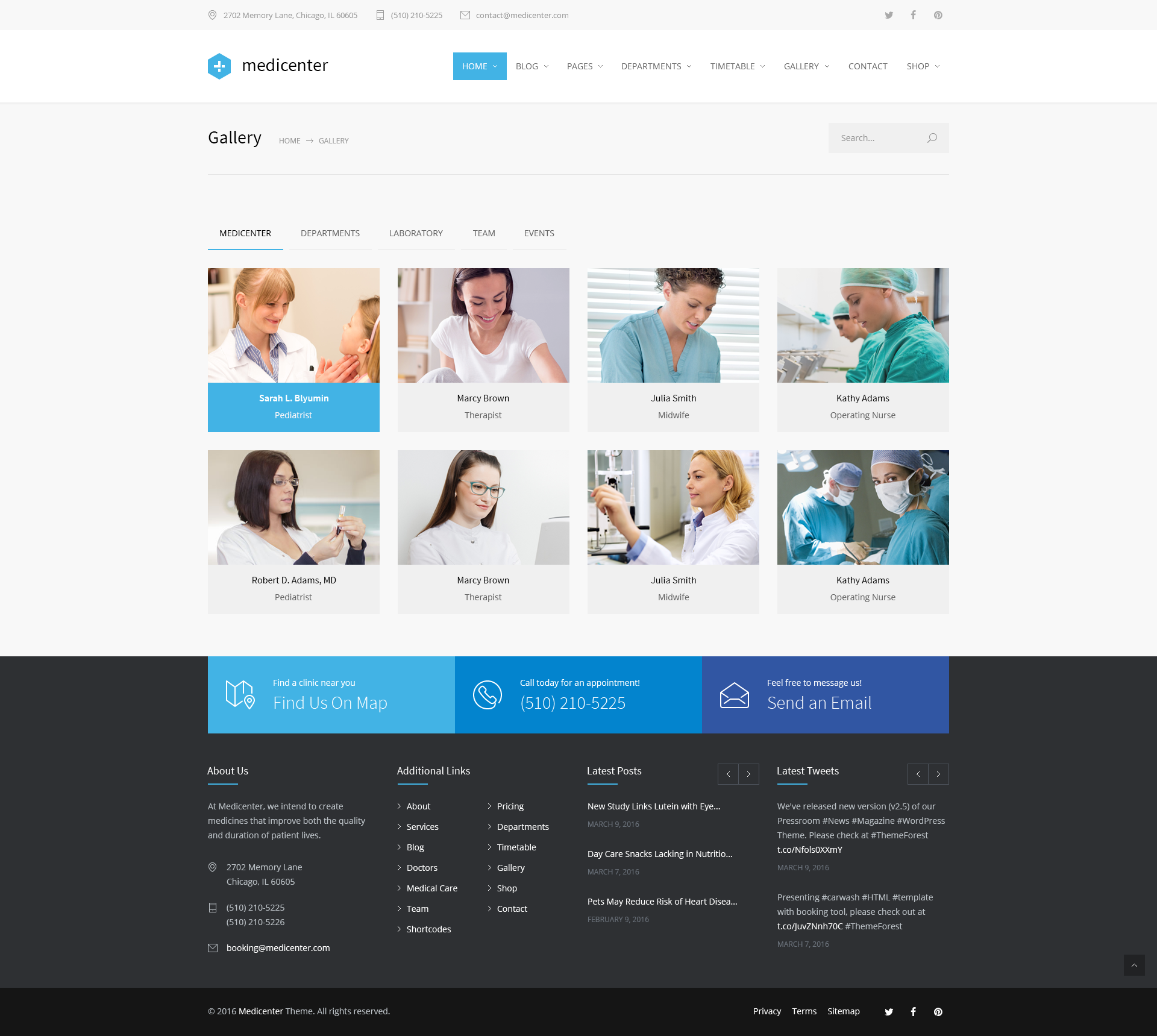This image is a detailed screenshot of a medical center's webpage. At the top, there's a pinned address: "2702 Memory Lane, Chicago, Illinois 60605," followed by a phone icon with the number +1 (510) 210-5225 and an envelope icon with the email address: contact@medicalcenter.com. On the far right, social media icons for Twitter, Facebook, and Pinterest are displayed.

The header outside the grey bezel features the company logo on a white background: a 3D hexagonal shape with a white cross inside. Next to the logo, in bold black lowercase letters, is the company name "MediCenter." To the right of this are navigation buttons: the first is a highlighted dark blue "Home" button with a white down arrow, indicating it is selected. Following this are black buttons for "Blog," "Pages," "Departments," "Timetable," "Gallery," "Contact" (without a down arrow), and "Shop."

Below, in bold black text, "Gallery" is displayed with a grey breadcrumb trail showing "Home" followed by an arrow pointing to "Gallery." Multiple sections are presented, with the first selected section highlighted by a blue underline under the title "MediCenter." Other sections in a faded grey-black mix include "Departments," "Laboratory," "Team," and "Events."

In the "Team" section, individual profiles are showcased in rectangles with subsections. The first selected profile is of Sera Lvyumin, a "Podiatrist." The image shows her checking a girl’s tonsils—Sera has blonde hair, is wearing a blue undershirt beneath a white medical jacket, and the girl has a light complexion, blonde hair with a pink bow, and a white shirt with a pink outline.

The next profile is Macy Brown, a "Therapist," depicted with short brown hair, a white t-shirt, grey pants, and a light complexion, smiling. Another profile features Julia Smith, a "Midwife," in blue scrubs, with curly short hair, and light skin, standing next to a window with drawn white blinds.

Additionally, there’s an image of Kathy Adams, an "Operating Nurse," shown with another nurse. Kathy is light-skinned and her hair is obscured by her scrubs. Another profile is Robert D. Adams, an "M.D. Podiatrist," in a medical jacket, glasses, with shoulder-length hair. There’s also Marcy Brown, again listed as a "Therapist," with teal-rimmed glasses, working on a gray computer.

Julia Smith appears again as an "M.W." with blonde hair, wearing a medical shirt and blue undershirt, working at a microscope in a lab. Lastly, there's an image of two doctors near an operating table with purplish-blue hair nets and white masks, wearing teal scrubs. The caption identifies the female as Kathy Adams, an "Operating Nurse."